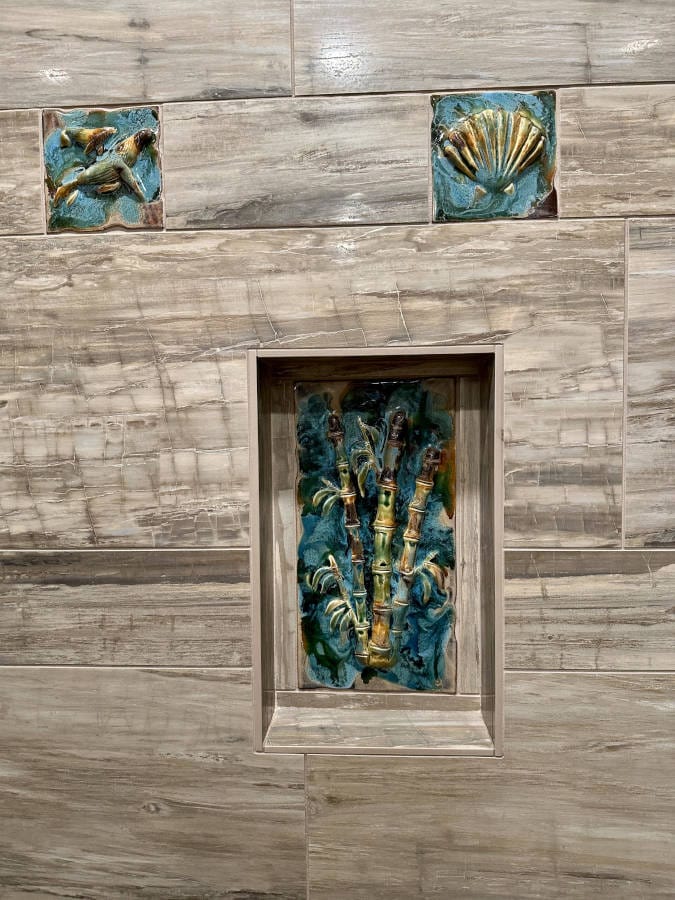This photograph, captured in portrait orientation, showcases a detailed and artistic indoor scene. The entire image is dominated by a wall comprised of horizontal boards in a light grayish cream color, resembling wood. The wall features intricate ceramic tile art insets that draw immediate attention.

Near the bottom center of the wall is a deeper, vertically oriented niche cutout. Inside this niche, a ceramic art piece depicts three vertical stalks of bamboo in a delicate array of light green, gold, and blue hues, set against a hand-painted, greenish-blue swirled background.

Above this niche, two smaller, square ceramic insets are mounted. The left square features an artistic portrayal of a pair of humpback whales, gracefully swimming through a similarly colored bluish-green background. The right square tile displays a seashell motif, with a fan-shaped shell in faded yellows and blues, convincingly crafted to appear aged and weathered by water. The entire composition is executed in a style that blends photographic realism with representational art, providing a sense of depth and texture to the handcrafted ceramic installations.